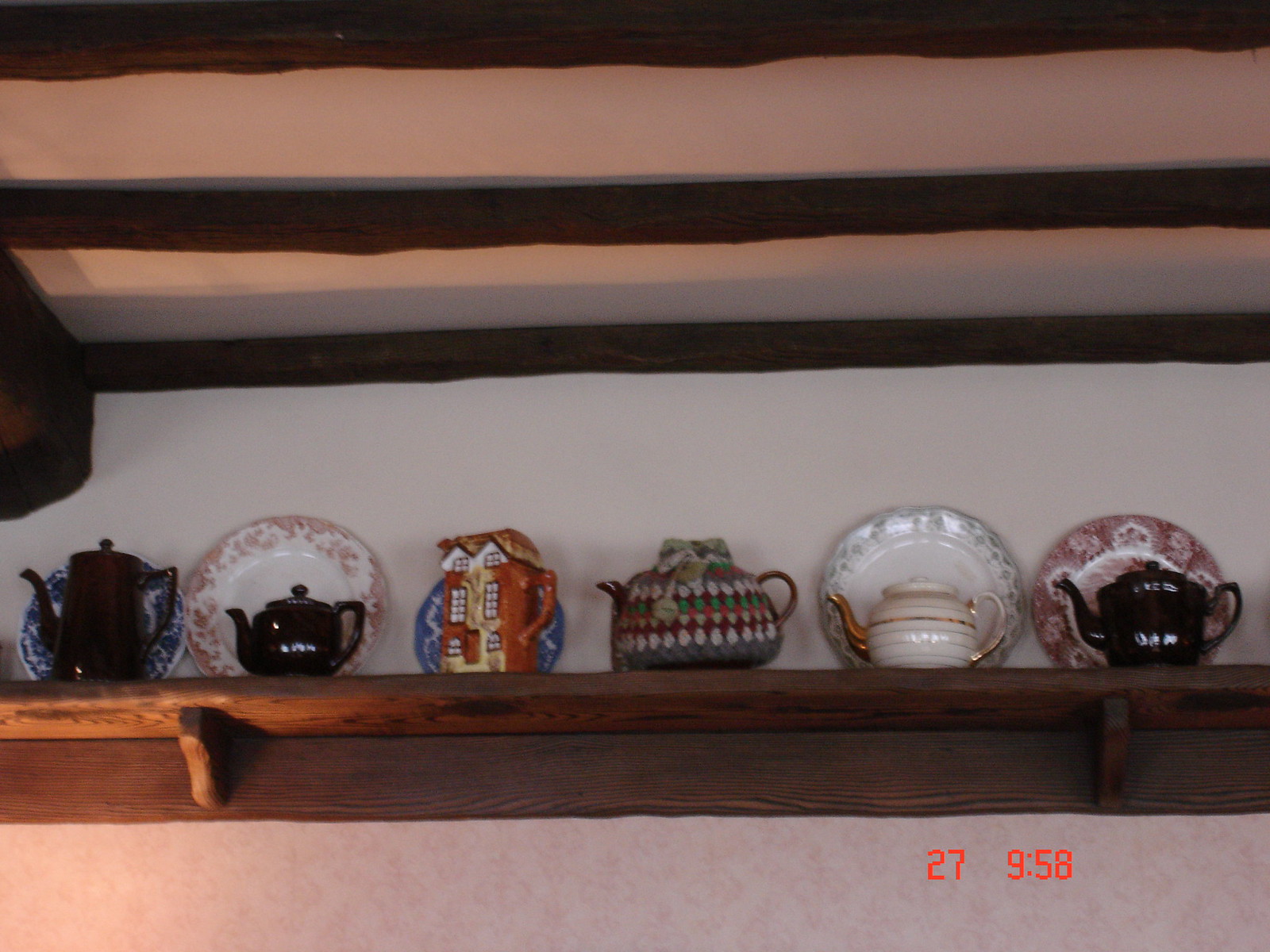The image captures an eclectic display of six teapots on a high, dark brown wooden shelf, set against a white-wall background. The ceiling features rough-hewn, exposed white beams with larger crossbeams, contributing to a rustic ambiance. The shelf itself is approximately 8 to 10 inches deep, with a thick, curved edge and supported by two sturdy bracketed supports. Below the shelf, there’s a hint of faint pink floral patterned wallpaper.

On the shelf, moving from left to right: a tall black teapot sits in front of a blue and white china plate; a shorter round black teapot is positioned in front of a white china plate with pink flourishes; a whimsical teapot designed to resemble a Swiss chalet has a blue and white china plate behind it; a teapot covered with what looks like a crocheted cozy sits without a visible plate; a delicate white teapot trimmed with gold has a white and gray plate behind it; and finally, another black teapot is placed in front of a pink floral-patterned plate. All the teapots' spouts are oriented towards the left. Near the bottom of the image, the numbers "27" and "9:58" are displayed in orange lettering, possibly indicating a time or date.